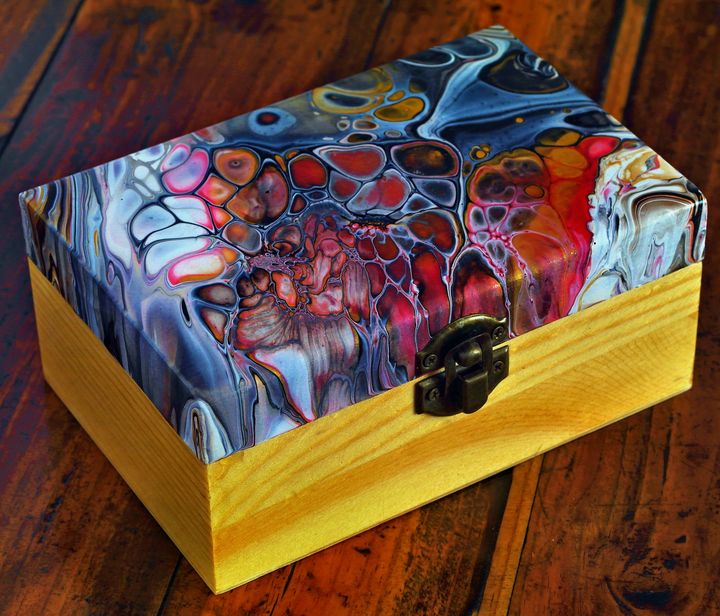This photograph captures a small wooden jewelry box sitting prominently on a dark-stained, slatted wood table that resembles a picnic table. The bottom half of the box is made from a lighter brown, beige-colored wood, contrasting with its metal clasp, which has a copper-like hue. The top of the box is intricately painted in an abstract, multi-colored design reminiscent of ink blots from the late 1960s to early 1970s. This vivid design features a spectrum of colors, including blues, oranges, reds, purples, whites, and blacks, creating a visually striking contrast with the more subdued wood tones of both the table and the box's base.